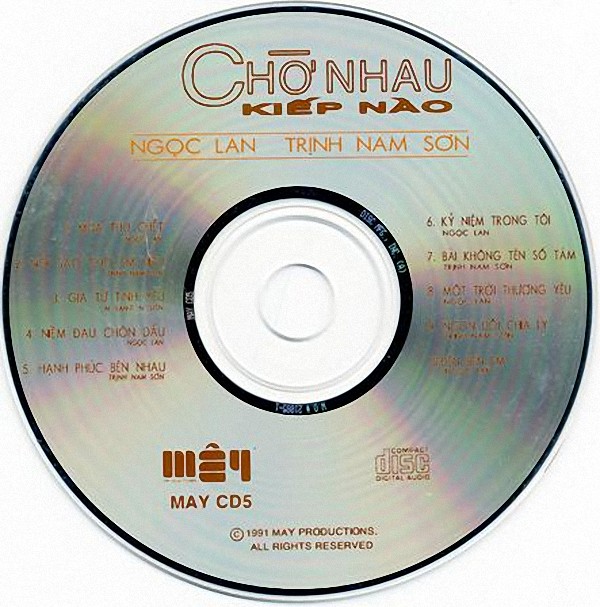The image is a close-up of a reflective, silver CD with distinct black borders around both the outer edge and the transparent inner circle. At the top of the CD, in red outlined letters, it reads "Chao, Han, Hu, Kiep, Niao". Below this, intersected by yellow lines, it states "NGOC Lan, Triumph, Nam, Sun". The lettering is primarily in light tan and dark brown, with additional text in orange.

On either side of the CD's center, there are listings of tracks, five on the left and five on the right, all in a non-English language. Some of the discernible track titles include:
1. [Unreadable]
2. [Unreadable]
3. Jio, Tao, Tung
4. Nim, Daung

Prominently displayed towards the bottom of the CD are several logos and text that include "May CD 5," and the phrase "compact disc, digital audio," alongside a copyright symbol reading "1991 May Productions, All Rights Reserved." The entire disc is highly reflective with various colored reflections and a clear outline, making the text and details stand out distinctly against the shiny background.